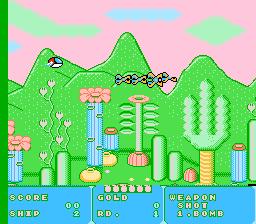This screenshot, evocative of a retro video game, features a surreal, vividly colored landscape. The sky is painted in an intense shade of pink, with an array of clouds in unusual colors: turquoise, green, and even a diamond-shaped one. The terrain below is a vibrant green meadow, rolling in bright, lively hues. In the foreground, various plants serve as decorative backdrops, including cacti and a variety of flowers. The flowers are diverse, some small and some large; they display shades of pink with blue bases, while others are purely white. High above, near the peak of a distant mountain, hovers a peculiar object—a square that melds white, blue, and red hues—adding to the fantastical atmosphere of the scene.